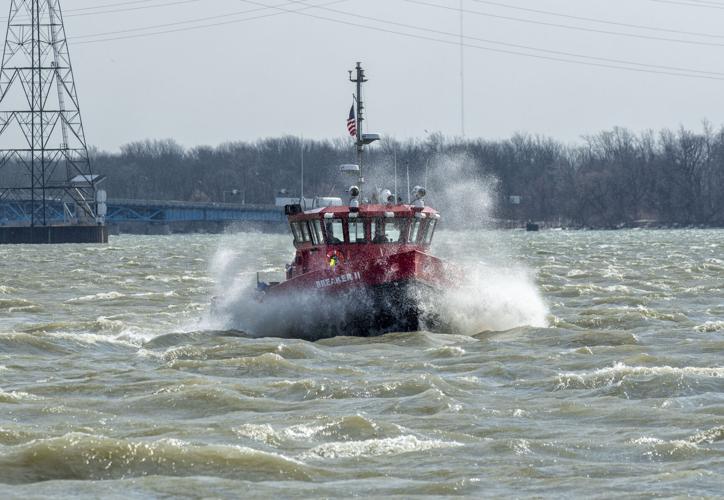The photograph features a red fire boat, reminiscent of a tugboat, swiftly navigating through choppy steel-gray waters dotted with white caps. The boat, positioned centrally and facing towards the viewer, displays an American flag flying at half-mast atop a long mast in the center over the wheelhouse. Surrounding the mast are various radar units, horns, and lights. The boat’s hull bears white lettering that is barely legible, and it sports black lining along the bottom. The water around the boat is turbulent, with white spray and mist indicating rapid movement. 

In the background, a dark, wintery tree line devoid of foliage stands under an overcast gray sky. Telephone poles and telegraph lines traverse the scene, adding to the bleak atmosphere. On the left side of the image, a tall wire tower extends out of the frame, while a steel-blue bridge spans the waterway, disappearing into the trees. The overall mood suggests a stormy day, with strong winds contributing to the rough water conditions.